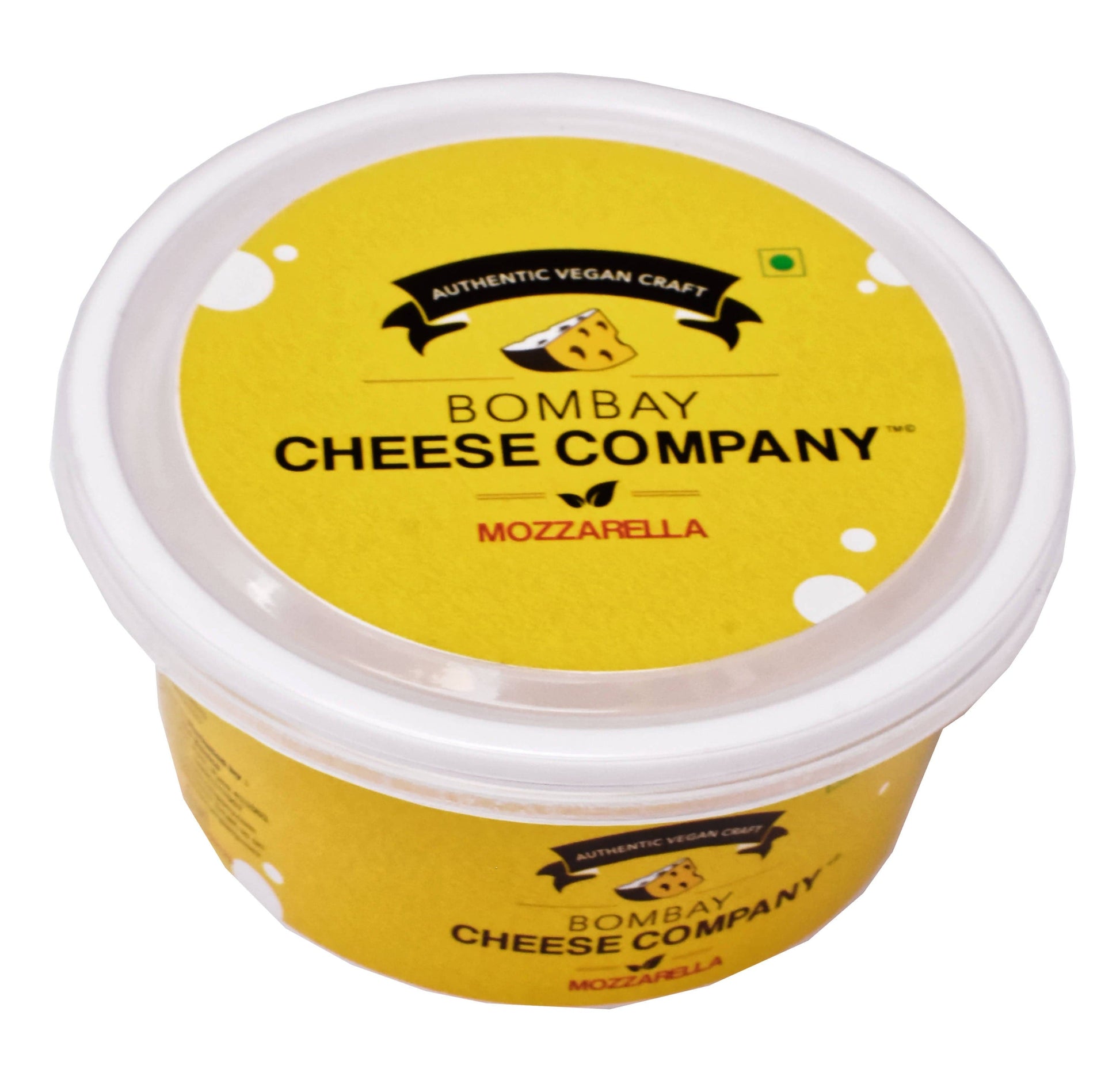The image features a circular plastic tub, characteristic of those used for margarine or whipped cream, prominently set against a stark white background, giving it a professional product photo appearance. The tub itself is yellow with a clear lid, adorned with a yellow circular label. On the label, a black banner reads "Authentic Vegan Craft," accompanied by an illustration of a hunk of cheese. Beneath this, in bold black text, it says "Bombay Cheese Company," followed by "mozzarella" in red lettering, bordered by a black leaf illustration as a divider. Although the tub’s side label replicates these details, it is less readable due to the high-angle perspective of the image, which emphasizes the top of the container. The scene suggests the tub contains a vegan mozzarella cheese alternative, aligning with the "vegan craft" and cheese imagery.